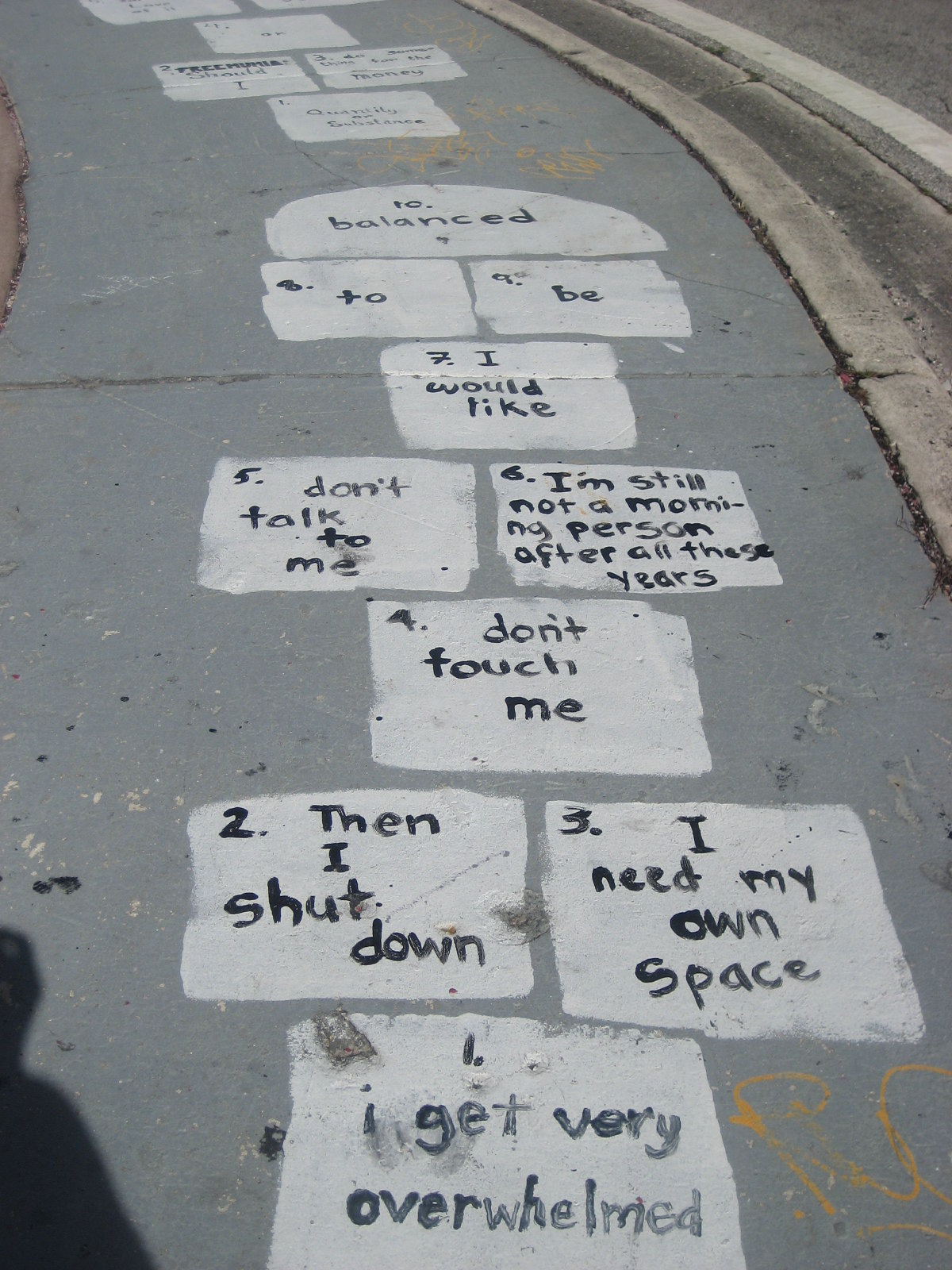This photograph captures a gray sidewalk painted with swirls of yellow and other spattered colors. The sidewalk features a meticulously crafted hopscotch game, artistically drawn not with chalk, but with white paint. Each segment of the hopscotch pattern follows the traditional format—one square, two squares, one square, and so forth—culminating in a semicircle at the top. Embedded within each square, in neat black handwriting, are numbers accompanied by a sequence of introspective phrases, forming a poetic narrative: 

1. I get very overwhelmed.
2. Then I shut down.
3. I need my own space.
4. Don't touch me.
5. Don't talk to me.
6. I'm still not a morning person after all these years.
7. I would like.
8. Two.
9. Be.
10. Balanced.

Adjacent to this artistic hopscotch is a second set, likely inscribed with different phrases, extending further down the curving sidewalk. The sidewalk itself curves gently to the left, and a curb borders the path, beside a strip of dirt or differently colored concrete. A faint shadow, possibly of the photographer, rests in the lower left corner, capturing a moment in the scene's vibrant yet reflective composition.